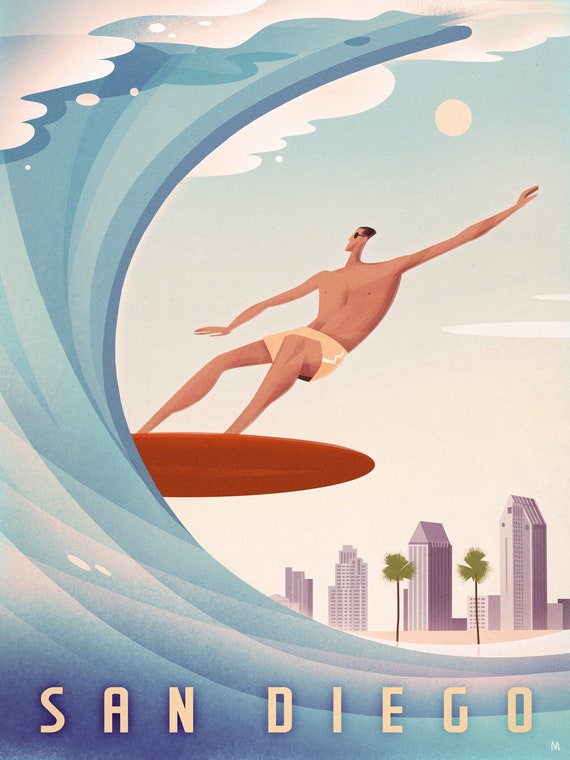The image is a vibrant animated poster showcasing a lively San Diego scene. Central to the illustration is a tanned surfer riding a massive, curving wave that sweeps from the bottom right to the upper left. The wave, depicted in shades of light blue and teal, dramatically engulfs him. The surfer, donned in light orange shorts, sunglasses, and sporting dark brown hair, has his right arm extended, emphasizing the dynamism of the ride. He is balancing on a brown surfboard which appears exaggeratedly stretched, mirroring his own disproportionately elongated body. Positioned mid-wave, his gaze is fixed intently on the impending swell to his left. In the backdrop towards the right, the serene beach is accented with a pair of palm trees and a cluster of four tall purple high-rises anchored at the bottom. Perched in the sky is a light yellow moon, juxtaposing the city's silhouettes. The scene is underpinned by the bold yellow text "San Diego" at the bottom, anchoring the composition and infusing it with a playful, sunlit atmosphere.